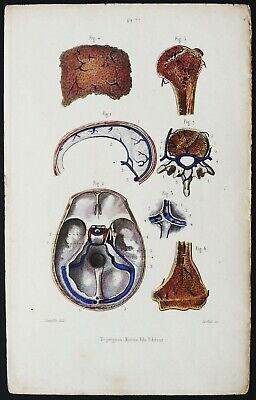The image features an illustration on an off-white, aged background, resembling an old page from a book. It displays various anatomical parts, likely bones and body parts, drawn with detail. The arrangement includes two items at the top row, followed by two more in the next row, a larger piece in the bottom left, and two smaller parts beside it. Among these illustrations, one appears to be a cracked, rectangularly curved piece that might be a skull fragment, another looks like the top part of a femur, one resembles a curved section with vein-like structures, and another part possibly depicts brain-like features. Additionally, there is an image that seems to be the top view of a skull, and another that might be the lower portion of a large bone, also resembling a femur. Each part is labeled with small, blurred figures and numbers (e.g., Figure 1, Figure 2, Figure 3) which are difficult to read. The entire illustration is bordered by a slim black line, and there is faint, illegible text at the bottom center of the page.